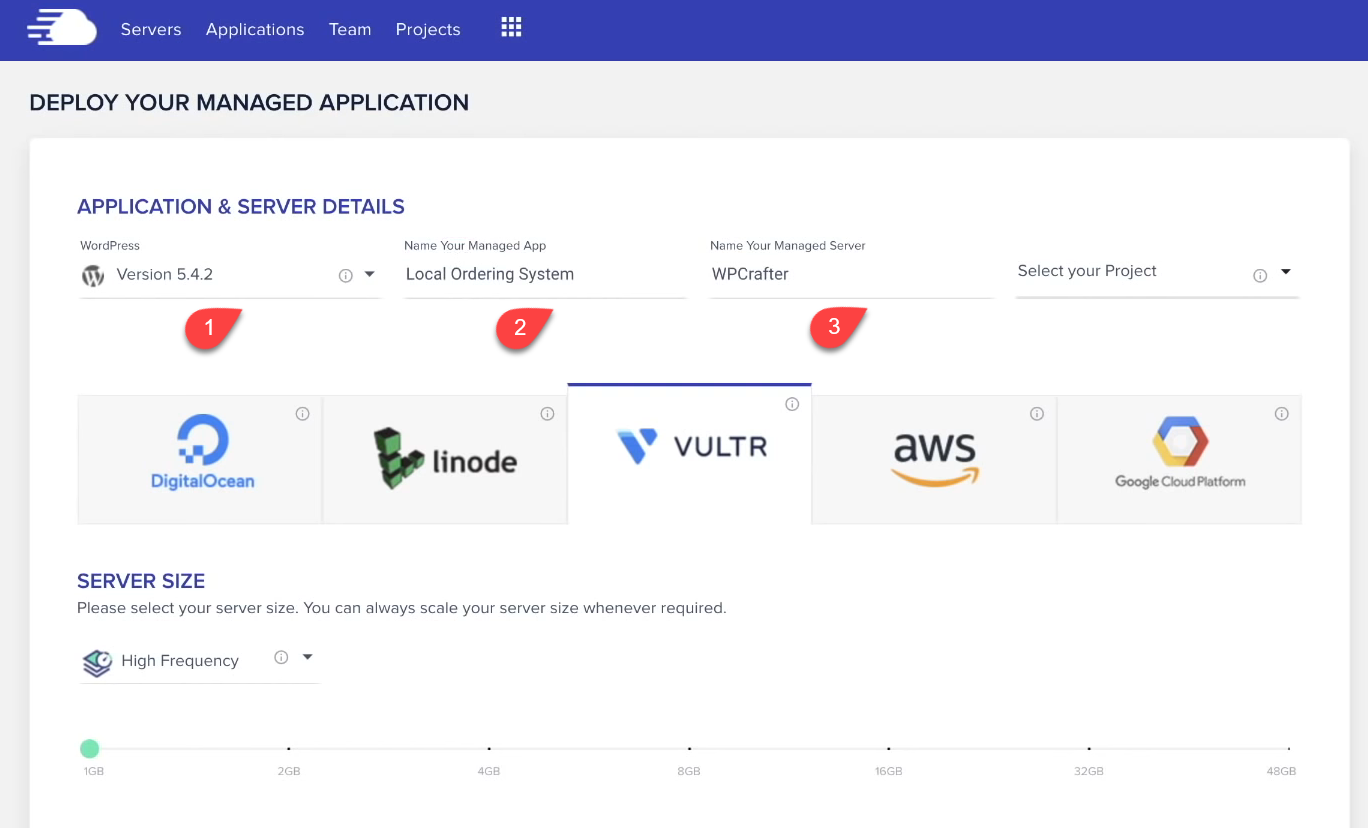**Category: Websites**

The website interface features a prominent blue header bar at the top, adorned with a white cloud icon accompanied by wind-like accents, signifying perhaps a weather-related theme or cloud management service. The header includes white text navigation options labeled "Servers," "Applications," "Team," and "Projects," followed by a grid-style menu icon on the far right.

Directly below the blue bar is a gray section, wherein black letters spell out the headline "Deploy Your Managed Application." This area acts as a separator preceding the main content section below.

The subsequent section is white and prominently displays the heading "Application and Service Details" in blue text. On the leftmost side, the interface lists "WordPress, version 5.4.2" next to a red raindrop icon containing the number one. Underneath it, the service provider is identified as "Digital Ocean."

To the right of this, the platform "Linode," spelled out as L-I-N-O-D-E, is represented with an arrangement of green blocks forming an 'L.' It has a red drop icon with the number two inside it.

Further to the right, "Vultr" (V-U-L-T-R), characterized by two blue lines, is accompanied by a red drop icon displaying the number three.

Overall, the webpage organizes deployment options for managed applications, listing service details and providers in a structured, color-coded interface.